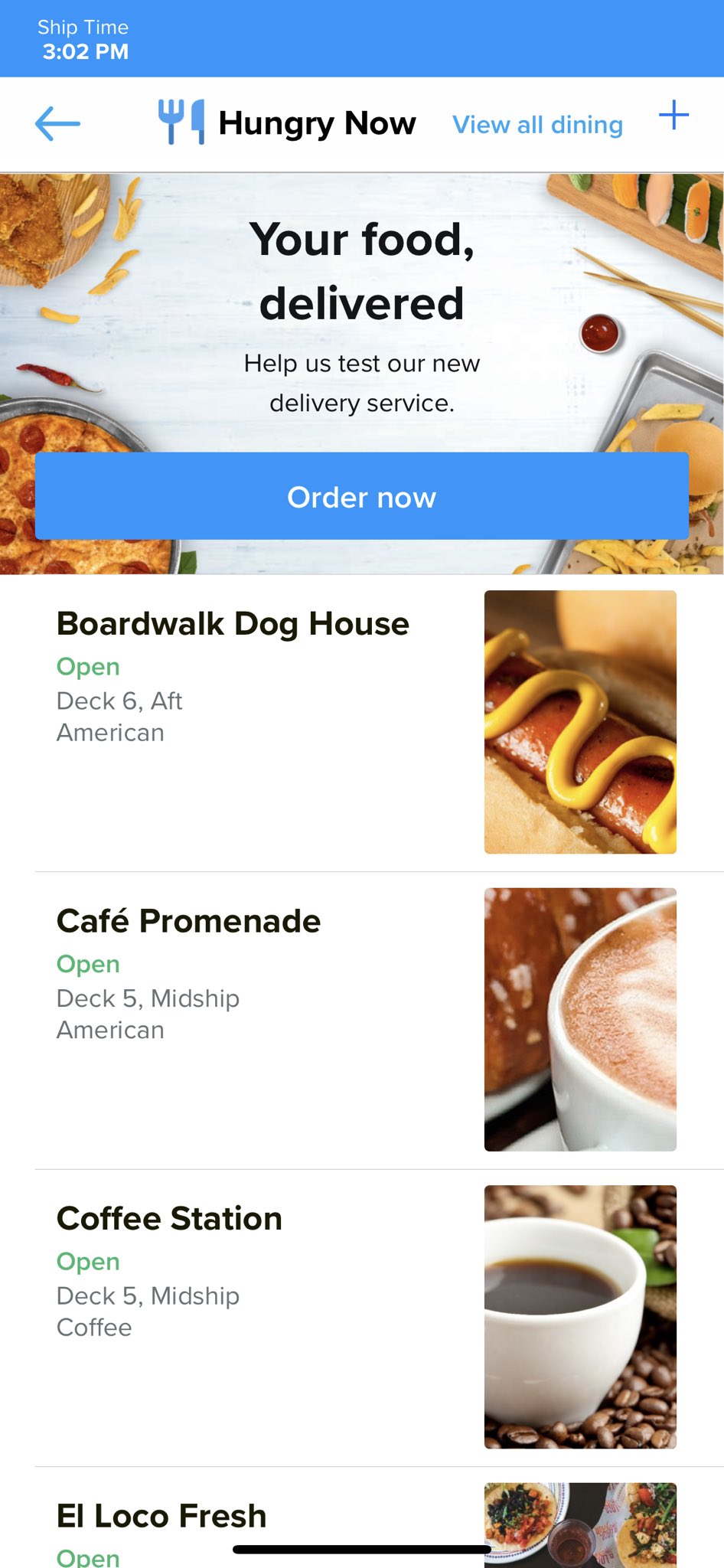This photograph is a detailed screenshot of a delivery app interface showing various food options and delivery notifications. The interface indicates that your food has been successfully delivered, with a prominent blue bar at the top of the screen displaying this status. 

At the top of the display, there is a blue bar that reads "Help us test our new delivery service." Below this message, a blue button labeled "Order Now" is also visible.

Several food items and dining options are listed on the screen. The first entry highlights a hot dog and custard, labeled "Open, Deck 6, American." The second entry lists the "Cafe Promenade" which is "Open, Deck 5, Midship, American." Another option, "Coffee Station," is noted as being "Open, Deck 5, Midship, Coffee." Finally, "El Boco Fresh" is included with an accompanying picture of some food.

All dining options that are currently available have the word "Open" written in green. Other informational text is displayed in a black font. There is also a promotional banner stating "Hungry now?" and another notification indicating "Your food has been delivered."

This detailed summary encapsulates the interface and the visual elements of the screenshot, providing a comprehensive overview of the screen's content.